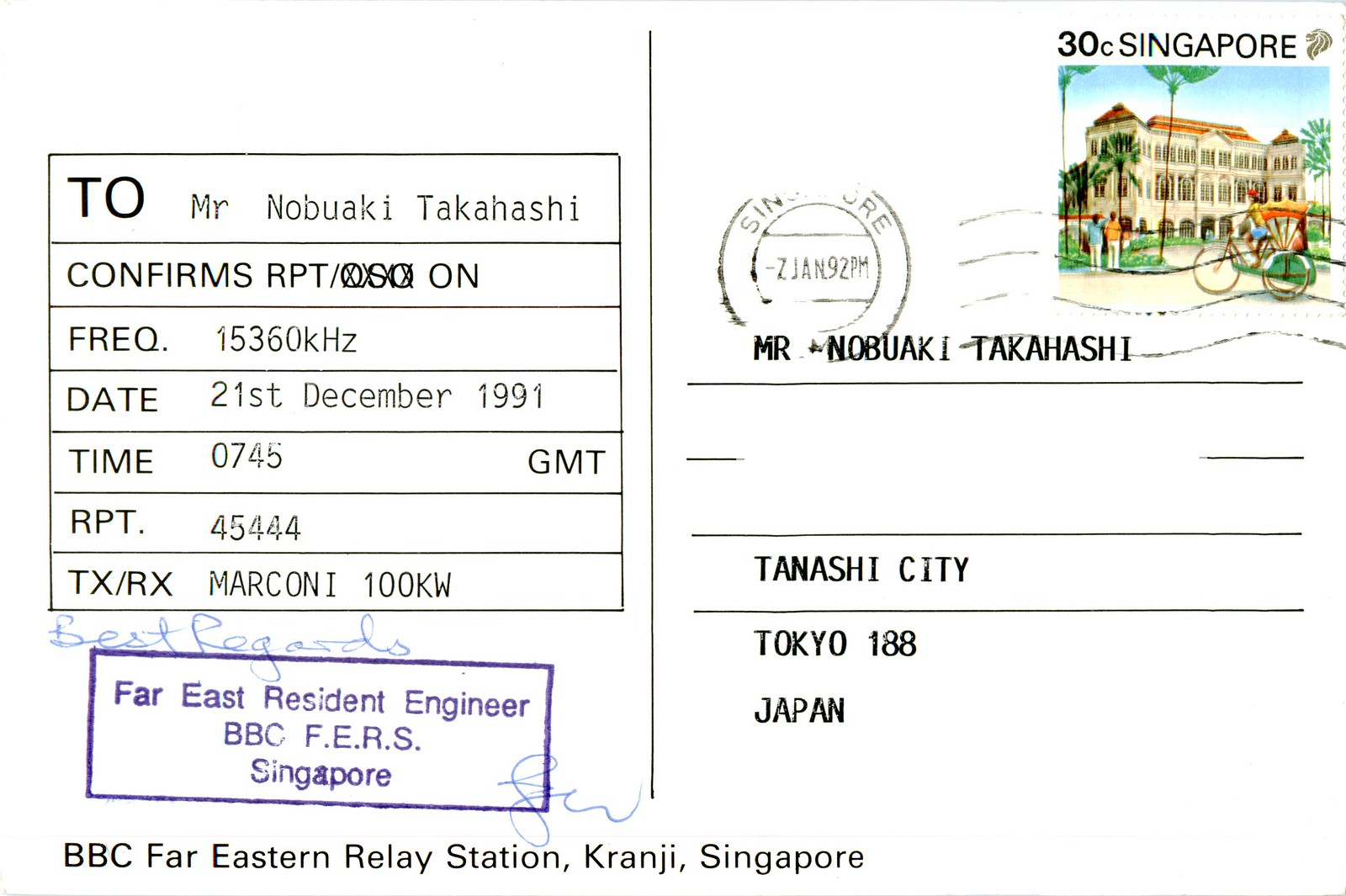This image depicts the back of a pristine white postcard, composed entirely of text and labels, meticulously aligning details. On the left side, it addresses Mr. Nobuaki Takahashi, noted in typewriter-like font. Below this, key transmission details are specified: "confirms RPT on FREQ 15360 KHz, date 21st December 1991, time 07:45 GMT, RPT 45444, TX/RX Marconi, 100 kilowatts." 

A stamp imprinted in purple ink reads "Far East Resident Engineer BBC F.E.R.S, Singapore." Handwritten in blue ink beneath these details, the message "best regards" adds a personal touch. The address "BBC Far Eastern Relay Station, Kranji, Singapore" is formatted at the bottom.

On the right side, a 30 cents Singapore stamp and postmark are affixed. Once again, Mr. Nobuaki Takahashi is identified, with his location noted as "Tanashi City, Tokyo 188, Japan." The unified details sketch a historical postcard meticulously noting significant radio transmission data and personal addresses.